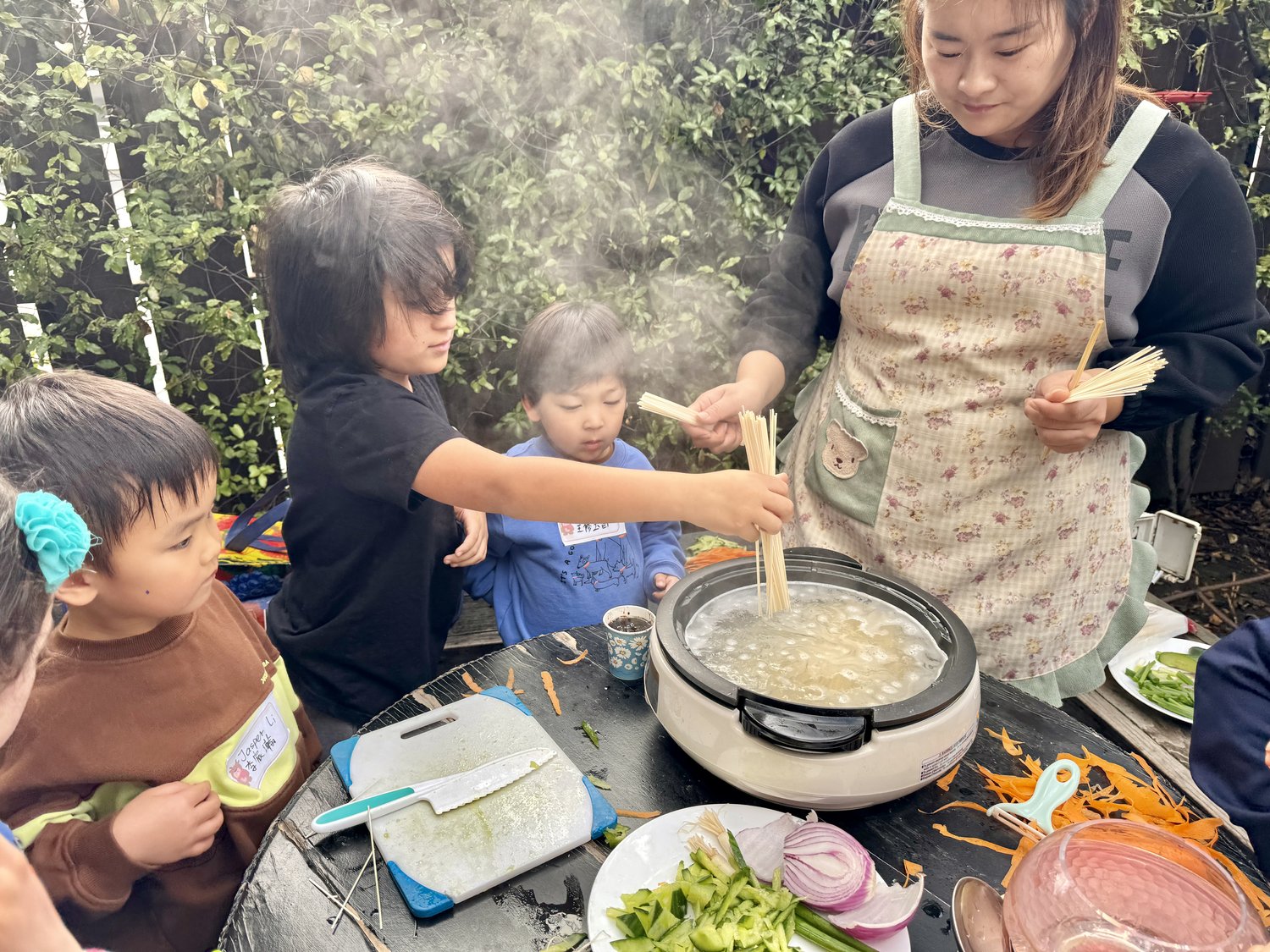The image captures a lively outdoor scene of a family preparing a meal together around a large, weathered black-painted round table with visible chips. In the center of the activity, a white crock pot with a black lid is boiling, and a young boy in a black shirt is carefully dropping uncooked spaghetti noodles into it. Standing to the right is an Asian woman, likely the mother, with her hair pulled back over her shoulder. She is wearing a light tan and white apron with green straps over a long-sleeved sweatshirt, both hands full of dry spaghetti. On the left, three more children—two boys and a girl with a blue bow in her hair—watch eagerly. One boy wears a blue shirt, and the other a red shirt. The table also holds a cutting board with a butcher knife, a plate with sliced red onions and celery, and shavings from carrots. An empty punch bowl sits in the lower right corner of the image. Behind this bustling family scene, dense green leaves form a natural, leafy backdrop, adding to the cozy, communal atmosphere of the photograph.